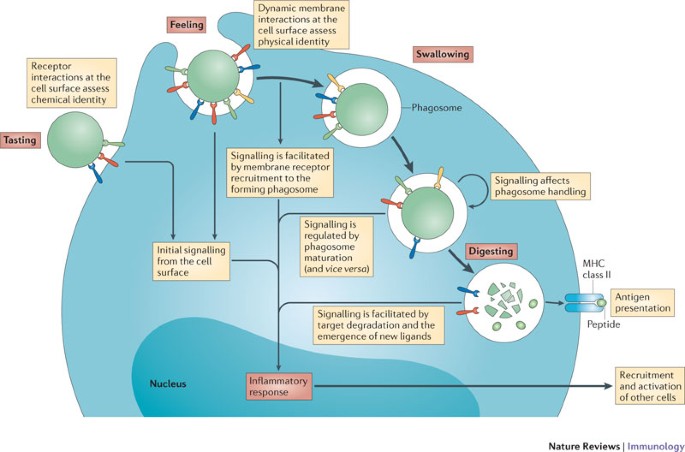This image is a detailed scientific diagram from Nature Reviews Immunology, predominantly illustrated in shades of blue and green, depicting various stages and processes within a cell. On the left side, it outlines the stages titled "Tasting," "Feeling," "Swallowing," and "Digesting," with descriptions of each process. 

Under "Tasting," it describes how receptor interactions at the cell surface assess chemical identity. "Feeling" involves dynamic membrane interactions at the cell surface to evaluate physical identity and mentions that signaling is facilitated by membrane receptor recruitment to the forming phagosome. The "Swallowing" section features an illustration of a phagosome and notes that signaling affects phagosome handling. The final stage, "Digesting," talks about antigen presentation and the recruitment and activation of other cells, emphasizing the inflammatory response present in the darker blue nucleus area at the diagram's bottom. This comprehensive depiction provides insight into the cellular process, highlighting crucial functional interactions and signaling pathways.